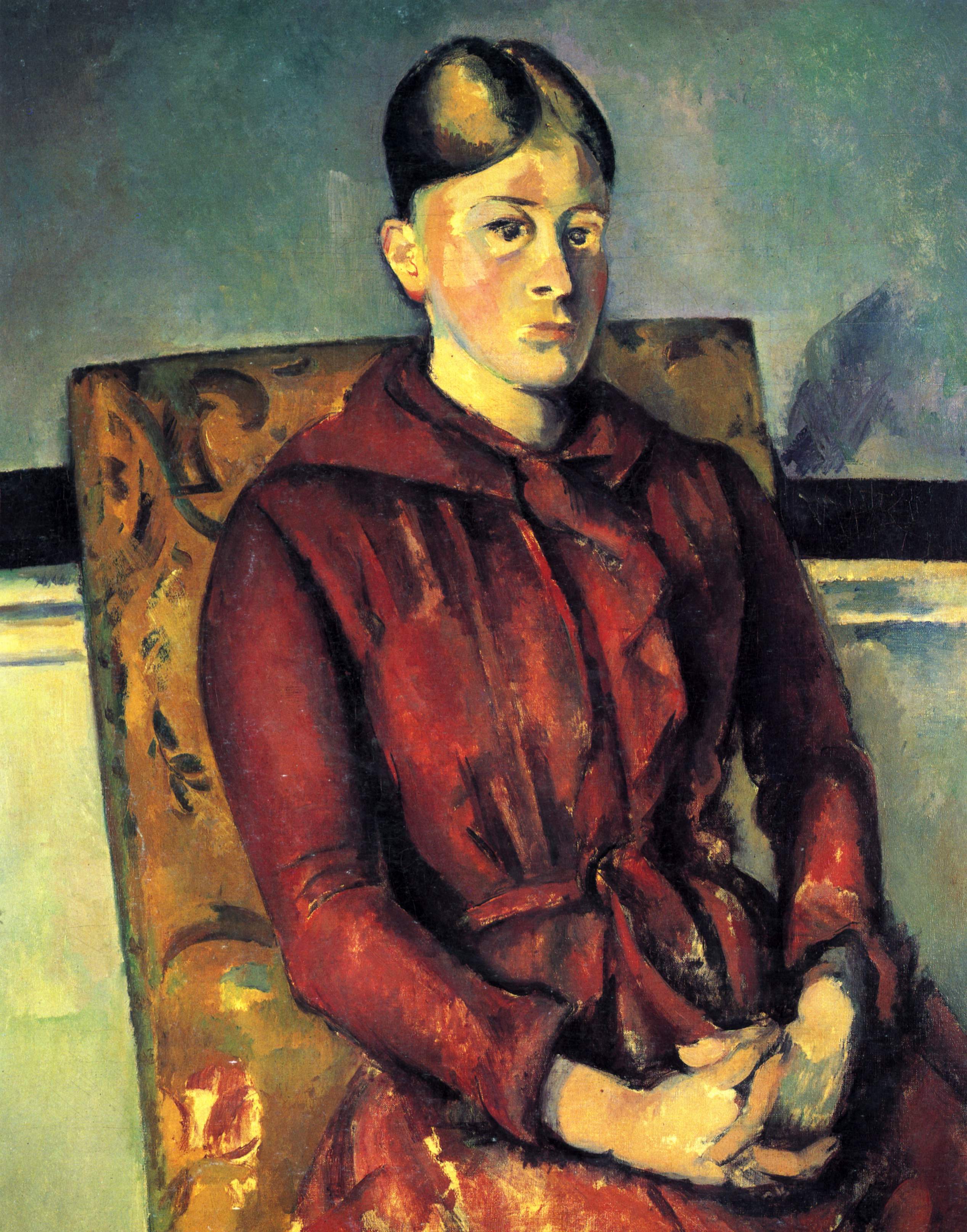This painting portrays a white woman seated in a brown upholstered chair. She is dressed in a long red dress with a sash tied in a knot at her waist. The woman has short brown hair, parted and slightly above her ears. Her facial expression is impassive, with large, dark, somewhat sad eyes and a closed, straight-lined mouth. She is looking slightly off to the side but also seems to be engaging the viewer with her gaze. 

Her hands are folded calmly in her lap. The background is plain and features a gray upper wall with some wainscoting detail and a lower section in a light bluish-green shade. The overall style of the painting leans towards the abstract, though it renders the subject's features and expression with clarity. Behind her, there is a mix of blue and green hues, and a prominent black line that may delineate different sections of the wall. The chair she is sitting on has hints of decorative red and green patterns, adding a subtle touch of intricate detail to the otherwise simple setting.